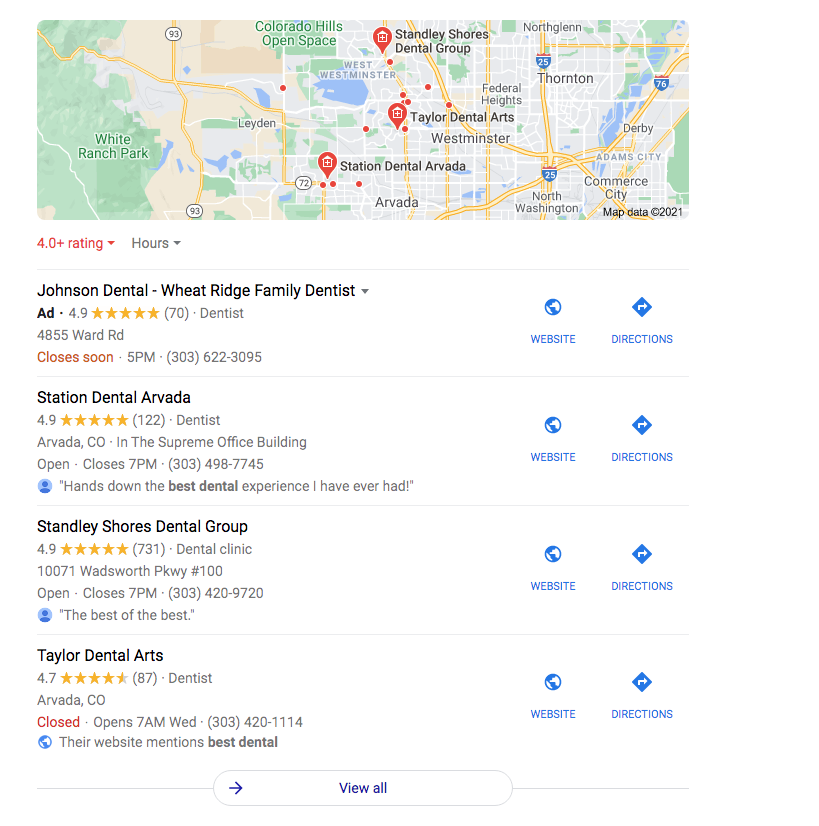The image is a vertically rectangular screenshot of a Google search result page focusing on local dental practices. At the top of the screenshot is a horizontally rectangular map, pinpointing three different locations. Directly beneath the map, on the left side, there is a red 4+ rating icon, indicating highly rated listings. Adjacent to this icon is an option to filter listings by their business hours.

Below this filter option, the search results begin with several dental practices listed as follows: Johnson Dental with a 4.9-star rating, Wheat Ridge Family Dentist with a 4.9-star rating, Station Dental Arvada with a 4.9-star rating, Stand Lee Shores Dental Group with a 4.9-star rating, and Taylor Dental Arts with a 4.7-star rating. To the right of each dental practice name, there are icons for accessing their website and getting directions. Centrally positioned at the bottom of the screenshot is a "View All" button, allowing the user to see more listings.